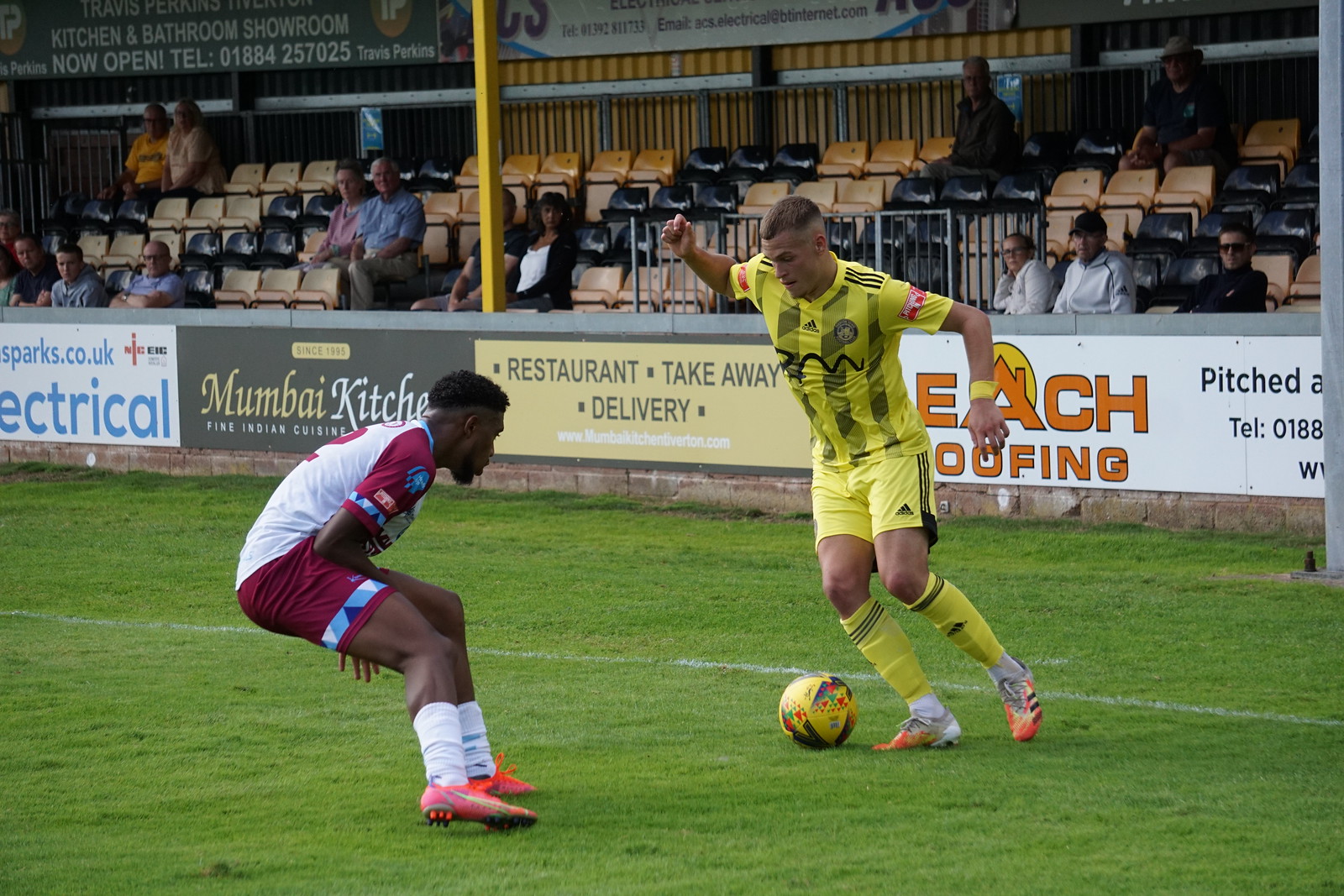In this outdoor soccer game photo, the focus is on two players engaged in a moment of play on a green grass field under sunlight. The player on the right, a white male with short hair shaved on the sides, is captured mid-action, poised to kick the yellow soccer ball. He is dressed in a bright yellow outfit featuring black stripes: a yellow jersey with black writing on the chest, yellow Adidas shorts with a black stripe, yellow socks, and orange cleats. To his left, the defender, an African American male, is crouched down, intensely watching the ball. He is wearing a distinctive dark red and white outfit with maroon sleeves on his white shirt, maroon shorts, white socks, and pink and orange cleats. The scene is set on a tidy grass pitch marked by a white line near the players' feet. In the background, a sparse crowd occupies about 20% of the yellow and black seats. The small stadium features various advertisements, including those from Moonby Kitchen, an Indian restaurant, a roofing company, and an electrical company, though the ads are partially cropped in the image. A short wall separates the seating area from the field.